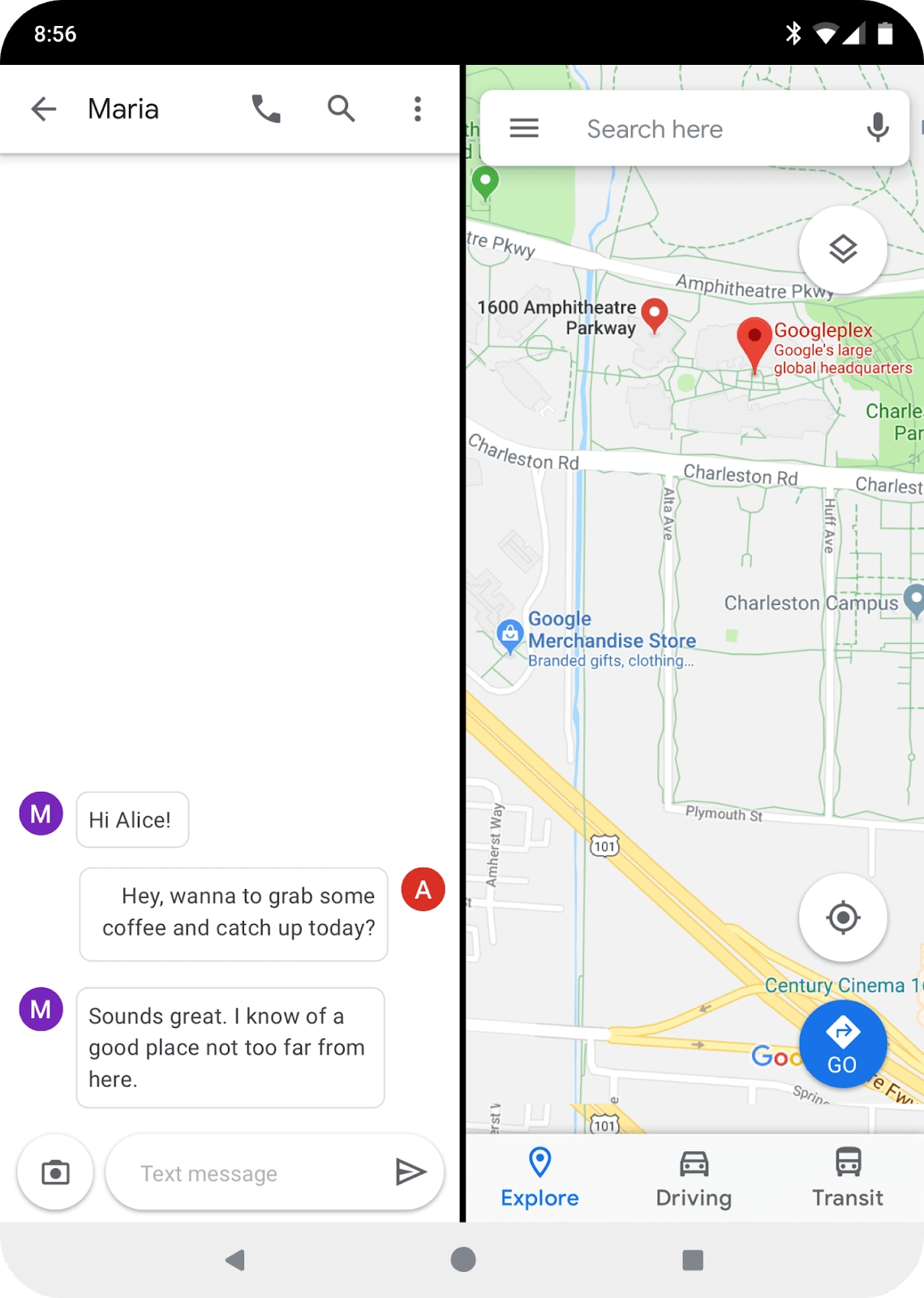In this screenshot of an Android phone, the display is divided into two main sections. The time at the moment of capture is shown as 8:56 AM in the top left corner, while the top right corner indicators show Bluetooth is active, the Wi-Fi connection is strong with approximately three bars, the cellular signal is solid, and the phone battery is largely charged.

On the left-hand side of the screenshot, there is a messaging conversation between two individuals. The user, presumably Alice, has received a message from Maria, saying "Hi, Alice." Alice replied with, "Hey, wanna grab some coffee and catch up today?" to which Maria responded enthusiastically, "Sounds great. I know of a good place not too far from here."

Meanwhile, the right-hand side of the screenshot shows the Google Maps interface open on the Explore page. Two points of interest are highlighted: the Googleplex and 1600 Amphitheater Parkway, indicating these are the selected locations. Although the specific city is not mentioned, it’s clear that these locations are in close proximity to each other.